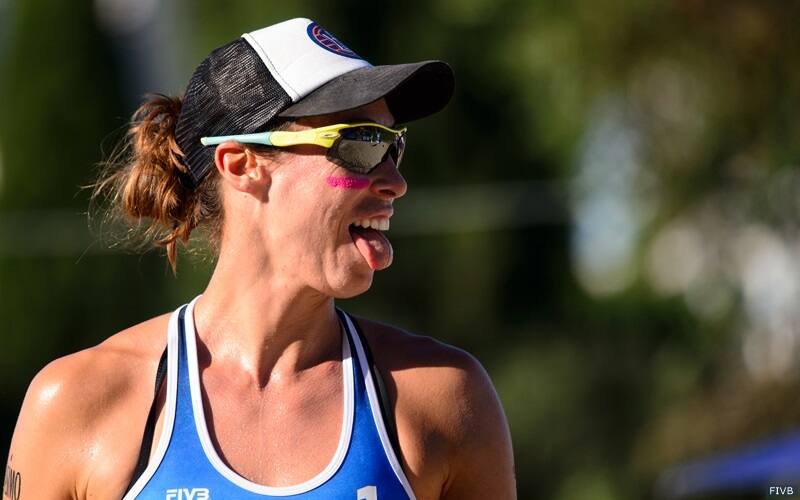The image depicts a Caucasian woman, possibly in her 30s, participating in a sports event, most likely volleyball. She is wearing black Oakley-style sports sunglasses with yellow and blue accents on the sides. Her attire includes a black cap with a white front, displaying an indistinct image. Her hair is pulled back into a ponytail, which is threaded through the back of her hat.

The woman is dressed in a fitted blue sports top, possibly a sports bra, trimmed in white. The number "5" and the upper part of another possible number "1" are visible on the top. She is photographed from the chest up, with her shoulders prominently shown. A tattoo is visible on her right arm, and pink lines are drawn under her eyes, adding to her sporty appearance.

Her mouth is open, and she is sticking out her tongue in a playful manner, perhaps celebrating or reacting to a play. She appears to be looking and slightly turning to the left from the viewers’ perspective. Her skin has a reddish hue, indicating exposure to sunlight. The background is green and blurred, suggesting an outdoor daytime setting, with bright reflections visible on her skin.